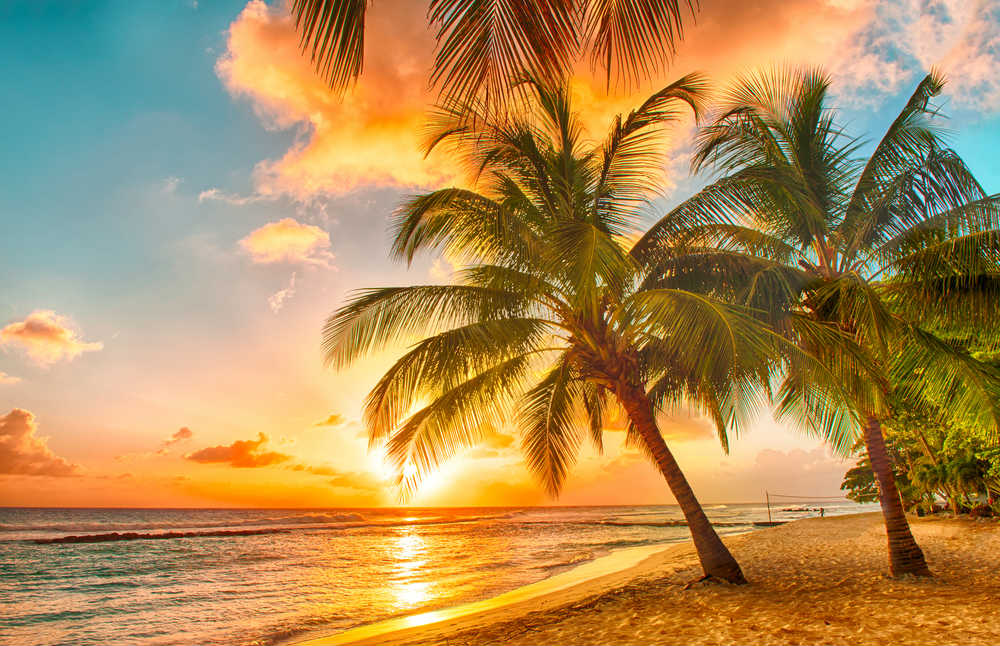A breathtaking photograph captures a serene beach bathed in the warm hues of a setting sun. Two almost identical palm trees, their thin leaves silhouetted against the sky, lean gracefully towards the calm, expansive ocean on the left. The golden sands stretch out to the right, with a volleyball net suspended in the distance between the two palm trees. The vibrant sunset paints the sky in striking shades of orange, pink, and yellow, illuminating white, puffy clouds. The sun, partly visible, casts a beautiful golden and orange glow over the water, which reflects the light, creating a mesmerizing blend of colors. Additional groves of palm trees dot the background, enhancing the tropical allure of the scene. The tranquil waves gently lap onto the shore, completing this picturesque and peaceful coastal vista.